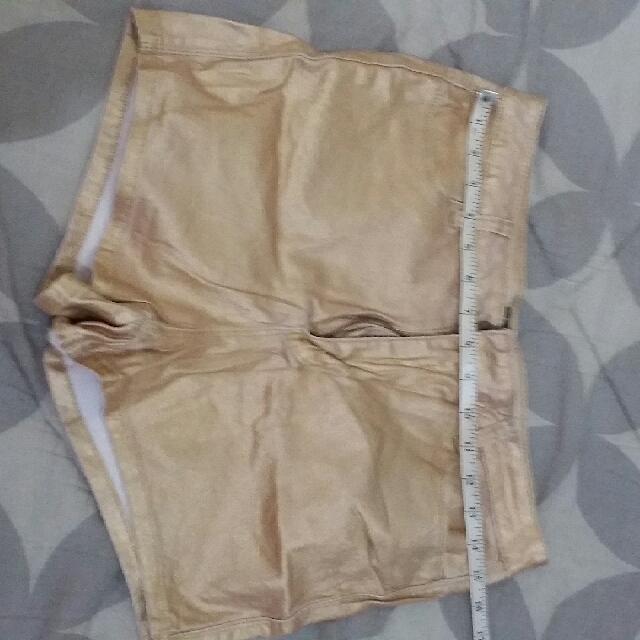This image depicts a pair of light brown, tan shorts neatly laid out on a bed with gray sheets, occupying the entire backdrop of the photograph. The shorts are centrally positioned, showing the zipper side facing up and the leg openings on the left, making their waist part directed toward the right. A tape measure, colored in an off-white or eggshell hue with visible but unreadable numbers, extends diagonally from the upper right of the image downwards. This scene, likely set in a bedroom, suggests the person photographing might be preparing to measure the shorts or their waist size, possibly considering outfit choices for the day. The photo is taken indoors and features a balanced color palette of grays, whites, and tans without any text overlay or distinguishing marks.